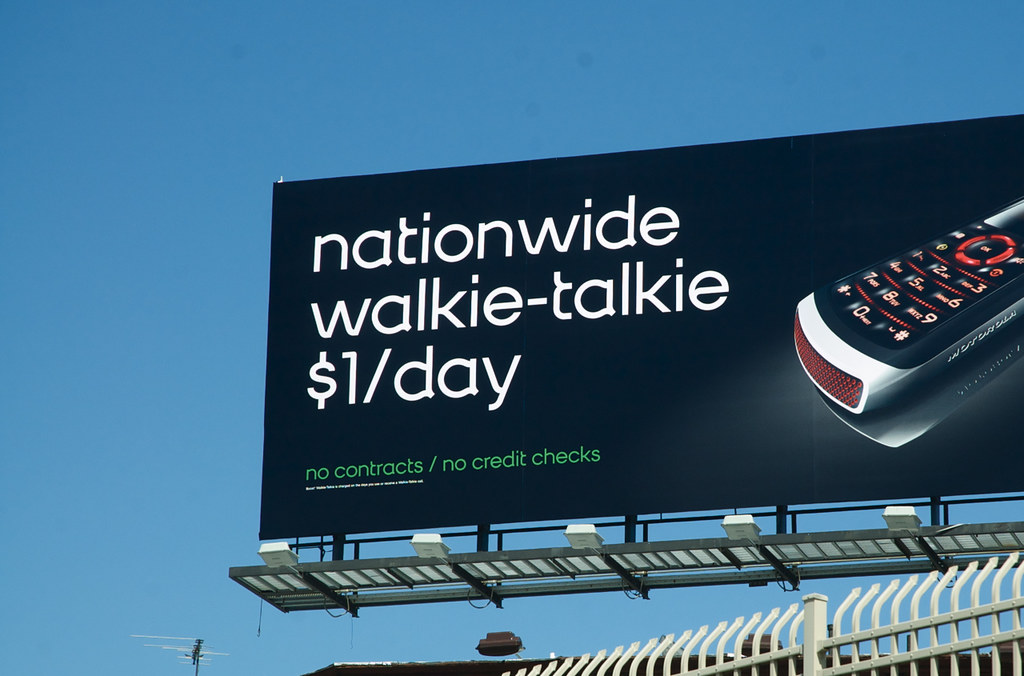Captured from an outdoor vantage point, this image presents an upward perspective revealing a striking blue sky as the backdrop. To the right, an antenna is visible, alongside the edge of a roof and a fence line suggesting the photo is taken from a rooftop. Dominating the scene is an imposing black billboard featuring a partial image of an old-school cell phone, reflecting light across its surface. The billboard advertises with the text: "Nationwide Walkie Talkie - $1 a Day. No Contracts. No Credit Checks," although it intriguingly omits any mention of the advertiser behind the promotion.